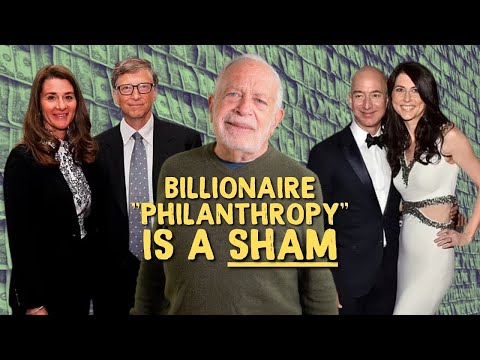The image is the cover of a YouTube video featuring the claim that billionaire philanthropy is a sham. Central to the image is an older man with gray hair and a beard, dressed in an olive sweater, who appears poised to present a video essay. Surrounding him are superimposed images of prominent billionaires: Bill and Melinda Gates on the left, and Jeff Bezos with his ex-wife on the right. The background is filled with cash, emphasizing the theme of money. At the bottom center, in bold yellow lettering, the phrase "billionaire philanthropy" is placed in quotes, with the word "sham" underlined, indicating a critical stance. This visually sets up the man's argument that billionaire donations are more about self-promotion than genuine altruism.